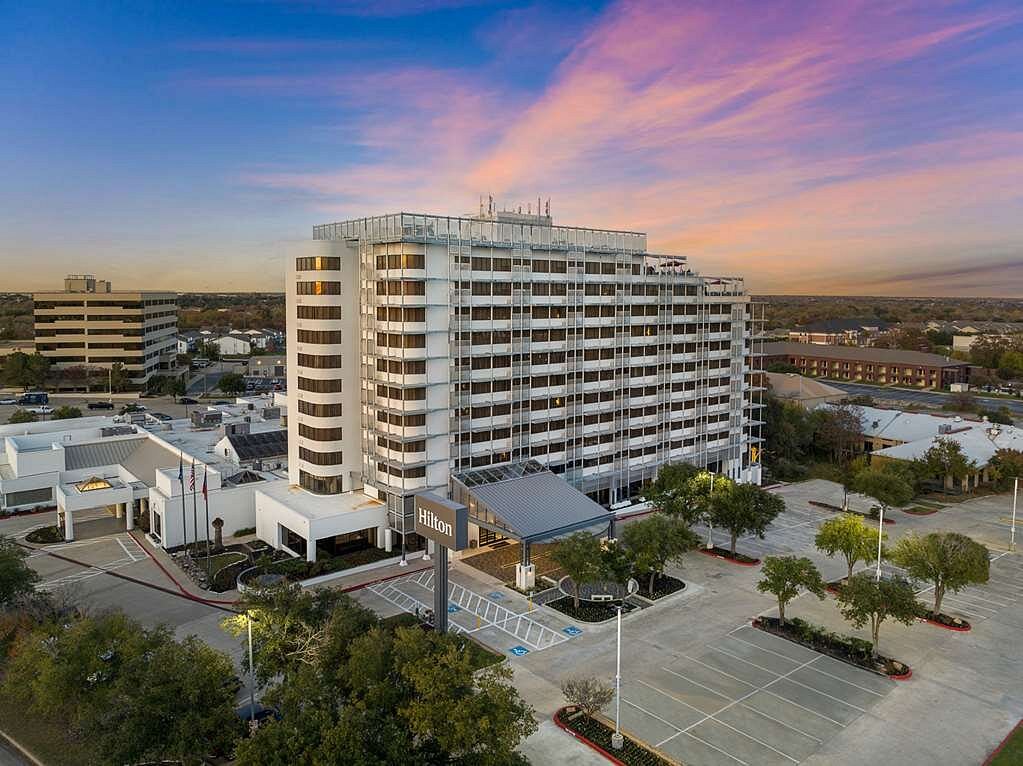The image depicts a large, multi-story white Hilton hotel building, prominently featuring silver lines that separate each floor and room. The building appears to be the focal point of the photograph, with a clear, gray Hilton sign visible in the empty parking lot below. The shot was taken from an elevated perspective, perhaps from a slightly lower or similarly high building, providing a nearly bird's eye view. The parking lot is completely devoid of vehicles, containing only streetlights and patches of lush green trees, some of which are positioned towards the bottom left of the image and within the lot serving as accessible parking spaces at the front. To the right of the hotel lies the expansive parking area, and to the left, a shorter tan office tower showcases a distinct architectural style. The sky is awash with vibrant hues of blue accented by pink, purple, and reddish-orange tones, indicating that the sun is setting, casting a serene and picturesque backdrop over the scene. The surrounding environment includes other buildings and houses, suggesting the hotel is situated in a less bustling, more suburban area.